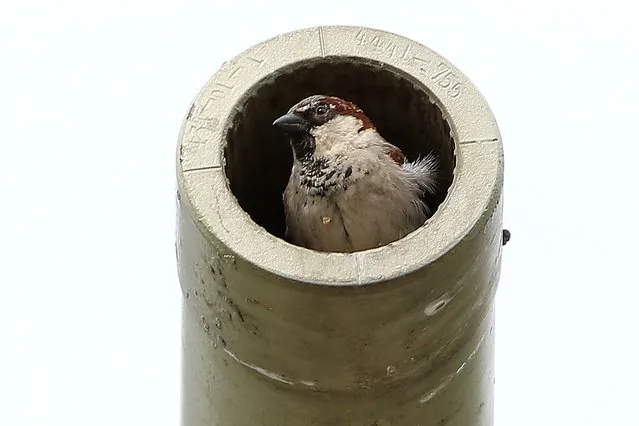In this detailed photograph, a small house sparrow is perched inside a circular beige or off-white pipe. The bird is peeking out of the pipe, looking to the left. With a brown crown, a black beak, and some black spots on its chest, the sparrow’s compact size allows it to fit snugly within the pipe. The pipe itself appears weathered, adorned with brown spots and dirt. There are distinct numbers, 444755, marked on the pipe, likely used for measurements. The background of the image is white, providing a stark contrast that highlights the bird and the pipe. The combination of the bird's natural colors—brown, black, and hints of white on its feathers—complement the rugged texture and appearance of the pipe, creating a striking visual.